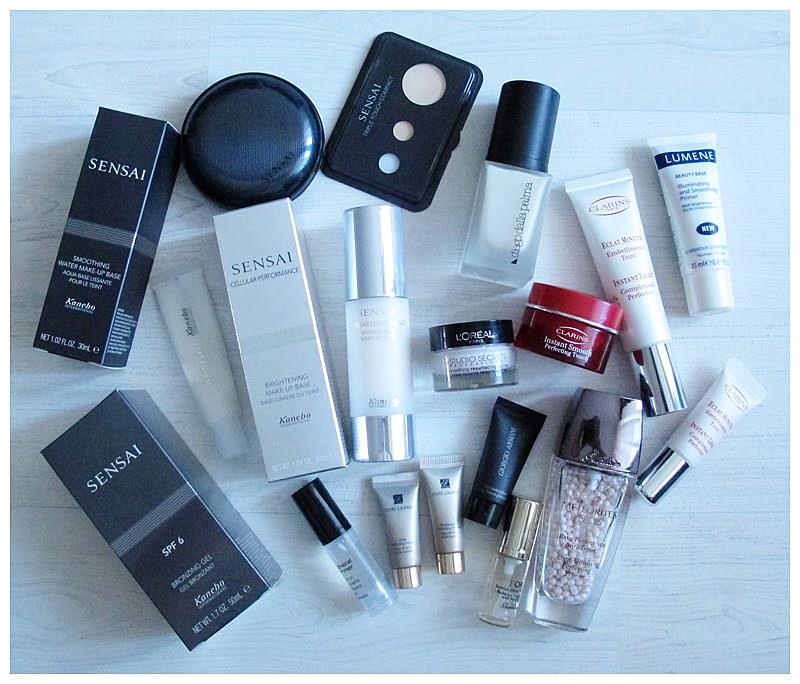On a white-ish wooden surface, which appears to be a vinyl plank floor, a diverse array of cosmetics is meticulously arranged. Prominent among them are skincare products from renowned brands such as Sensai, Luminae, Clarins, and L’Oreal. The collection includes several Clarins items, known for their premium skincare benefits. An SPF 6 sun protection product, providing minimal defense against UV rays, is also present. 

The assortment features a variety of formats, including boxed items, compacts, and tubes. The tubes range in size from small, portable ones ideal for a purse, to larger, more substantial containers. Two notable compacts are visible: one blue, and the other black, the latter revealing a trio of blush shades in blue, peach, and a tan/off-white hue. Among the items is an intriguing container with beads, whose purpose remains unclear.

The predominant color theme here is white, especially among the tubes, interspersed with blue accents. This well-rounded collection embodies both everyday essentials and specialized skincare treatments, highlighting the meticulous curation behind this display.